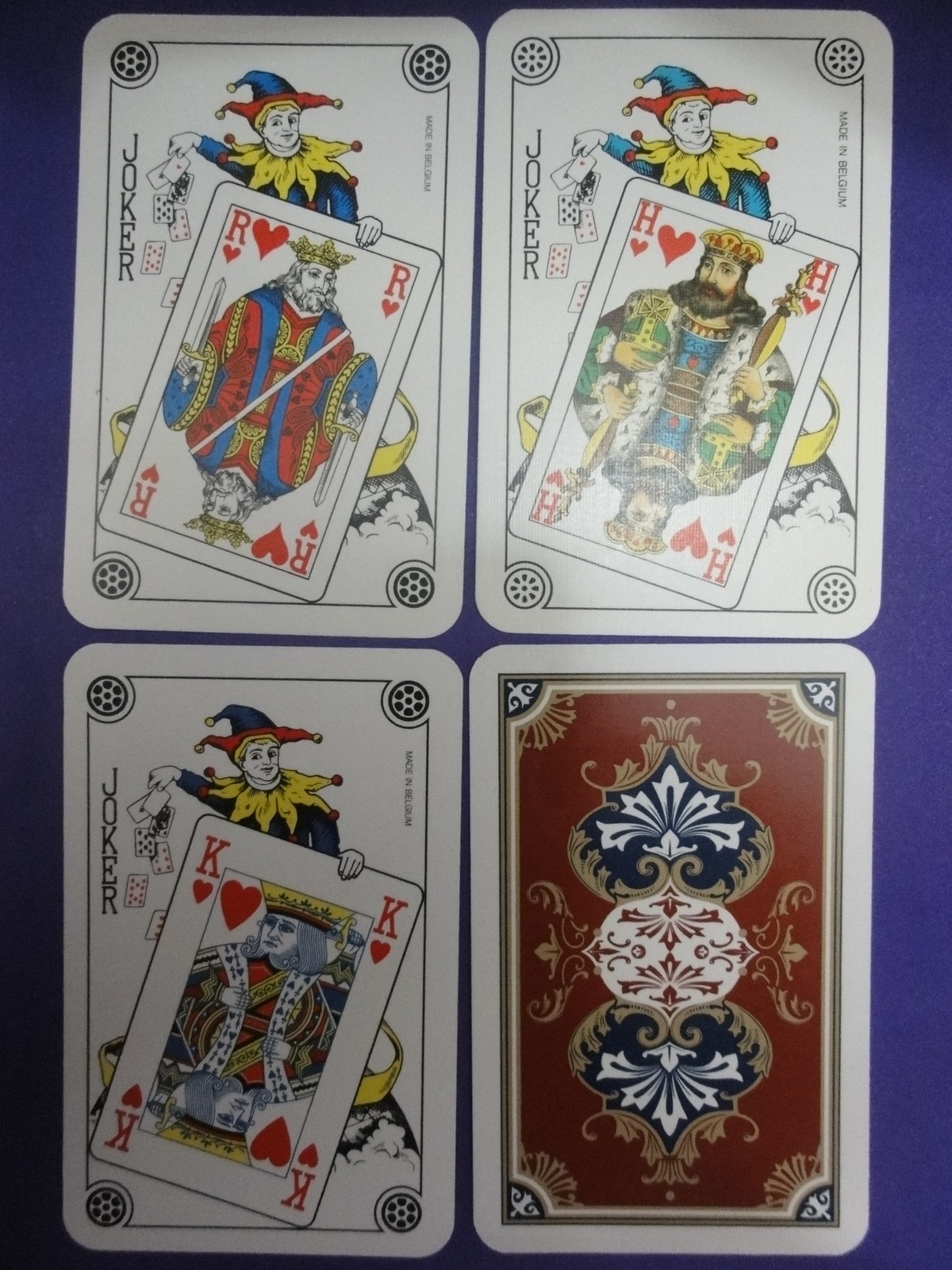This photograph showcases four playing cards, three of which are face-up while the fourth is face-down, revealing its intricate back design. The three face-up cards all feature a Joker character, each depicted holding a different King card. The Joker in the top left corner is dressed as a clown or juggler, presenting a King of Hearts card marked with an 'R' and a heart symbol. The Joker in the top right corner holds a King card labeled with an 'H' and a heart symbol. The Joker in the bottom left corner also presents a King of Hearts, distinct from the other two. The face-down card in the bottom right corner displays a Victorian-style pattern in shades of mauve, blue, gold, and white, adorned with intricate floral designs.